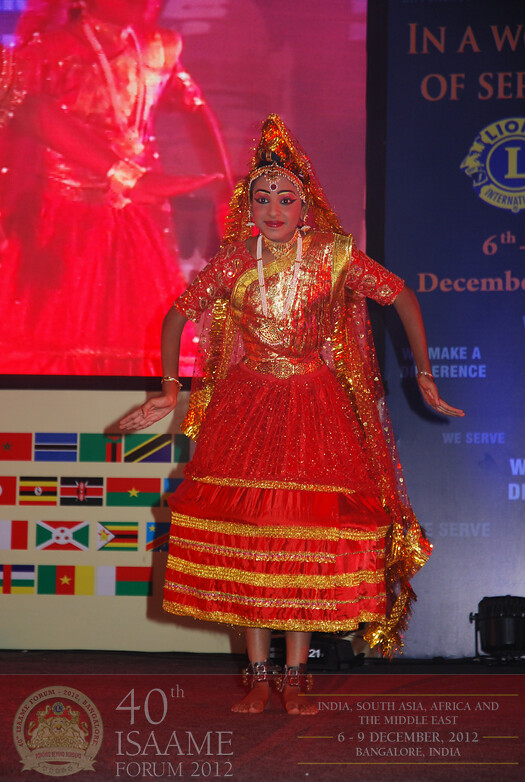A woman stands gracefully on stage, exuding elegance in an ornate costume. She is framed by a backdrop adorned with vibrant flags, enhancing the theatrical atmosphere. Her attire is a resplendent red and gold dress that glistens under the stage lights, complemented by an elaborate headdress that adds a touch of regal splendor. Barefoot, she wears delicate anklets that jingle softly with her movements. She strikes a poised stance, with arms extended to her sides and slightly bent, her fingers and hands flexed toward the ceiling in a gesture of artful expression. Her gaze is steady and intent, directed out into the audience, captivating their attention with her commanding presence.